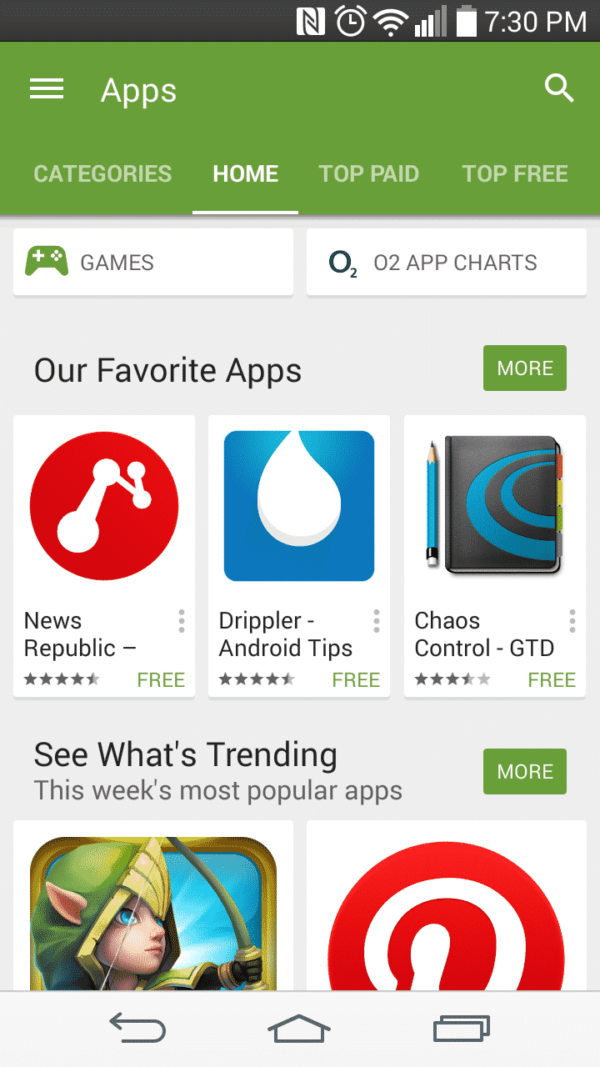Screenshot from a mobile phone displaying an app store interface. At the top is a gray status bar featuring several white icons: an "N," a white square, an alarm clock, a Wi-Fi signal, a mobile signal, and a battery indicator. The time is displayed as 7:30 p.m. Below the status bar, there is a green rectangle with three horizontal white lines and the word "Apps" to the left, and a magnifying glass icon to the right. 

The next section features navigation options: "Categories," "Home," "Top Paid," and "Top Free," with "Home" currently selected and underlined in white. 

Beneath this, a white rectangle displays a green controller icon with the word "Games," followed by another white rectangle labeled "O2 App Charts," indicated with a subscript "2" icon next to a zero. 

The subsequent gray background area contains the text "Our Favorite Apps" in black font, with a green "More" button to its right. Below this, three listed apps are shown: "News Republic," "Drippler," and "Chaos Control." 

Finally, the section concludes with the prompt "See What's Trending: The Week's Most Popular Apps."